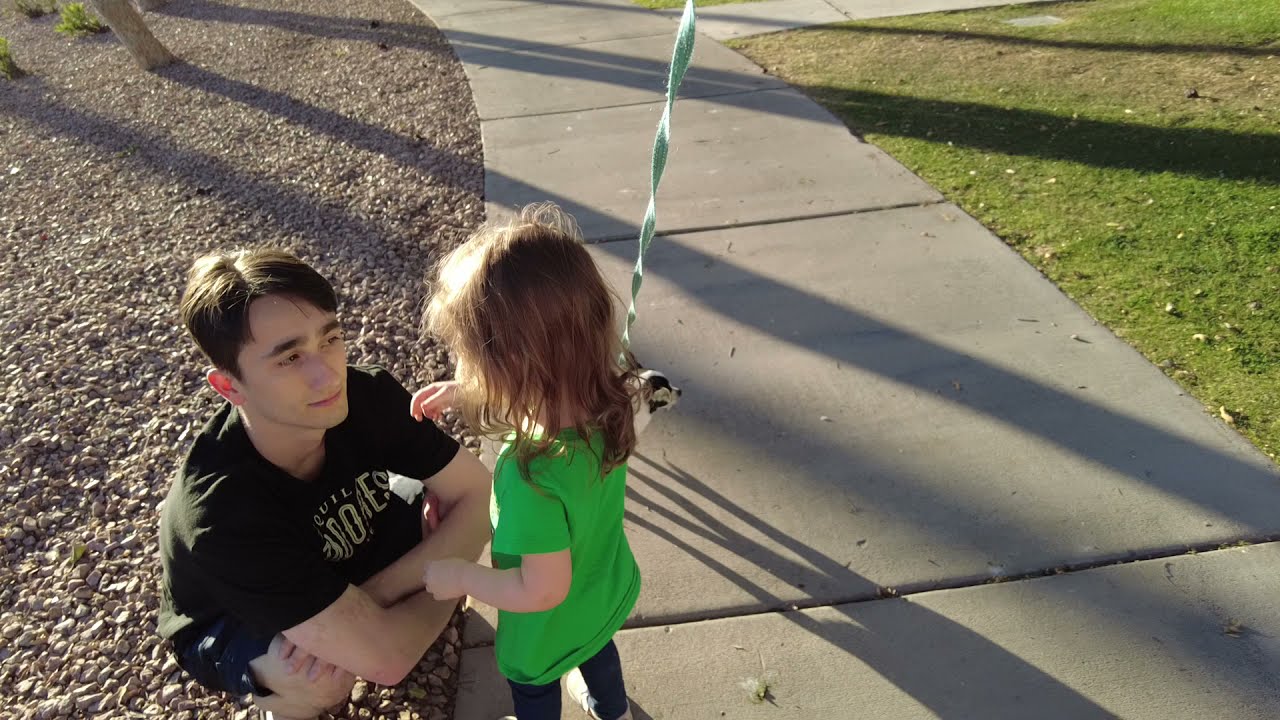In this photo, a man and a young girl are interacting on a sidewalk in what appears to be a residential area. The man, who has black hair swept to the side, is squatting down to be at the child's eye level. He is positioned slightly off the sidewalk on a rocky area to the left, and he is wearing blue shorts and a black t-shirt with some indistinguishable lettering on it. The girl, standing on the sidewalk, is dressed in a green t-shirt and blue jeans. She has shoulder-length hair and seems to be reaching towards the man with her right hand. A small dog, partially hidden behind the girl, is attached to a leash that the girl might be holding. To the right of the sidewalk is a grassy area, with another sidewalk veering off to the right, and the background features a few trees. It appears they are sharing a moment during their walk, enjoying each other's company.